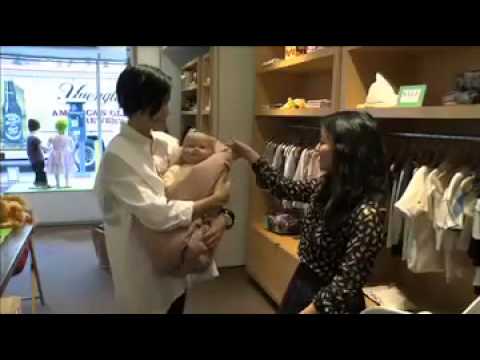The screenshot appears to be taken from a video clip inside a brightly lit baby clothing store. In the upper left corner of the image, the store's windows reveal a sunny day outside with writing on the glass and two children's mannequins displayed: a girl with a bright green cap and light-colored dress, and a boy with a dark outfit and black hat. The focus is on two individuals in the foreground. On the left, a man with slicked-back black hair, dressed in a white long-sleeve button-up shirt, holds a baby (possibly a doll) wrapped in a thick pink blanket. To his right stands a woman with long black hair, dressed in a black and white patterned top and black pants, possibly an interviewer or store employee. She is extending her right arm toward the back of the baby's head. The background includes racks of baby clothing, further indicating the setting is indeed a baby clothing store.